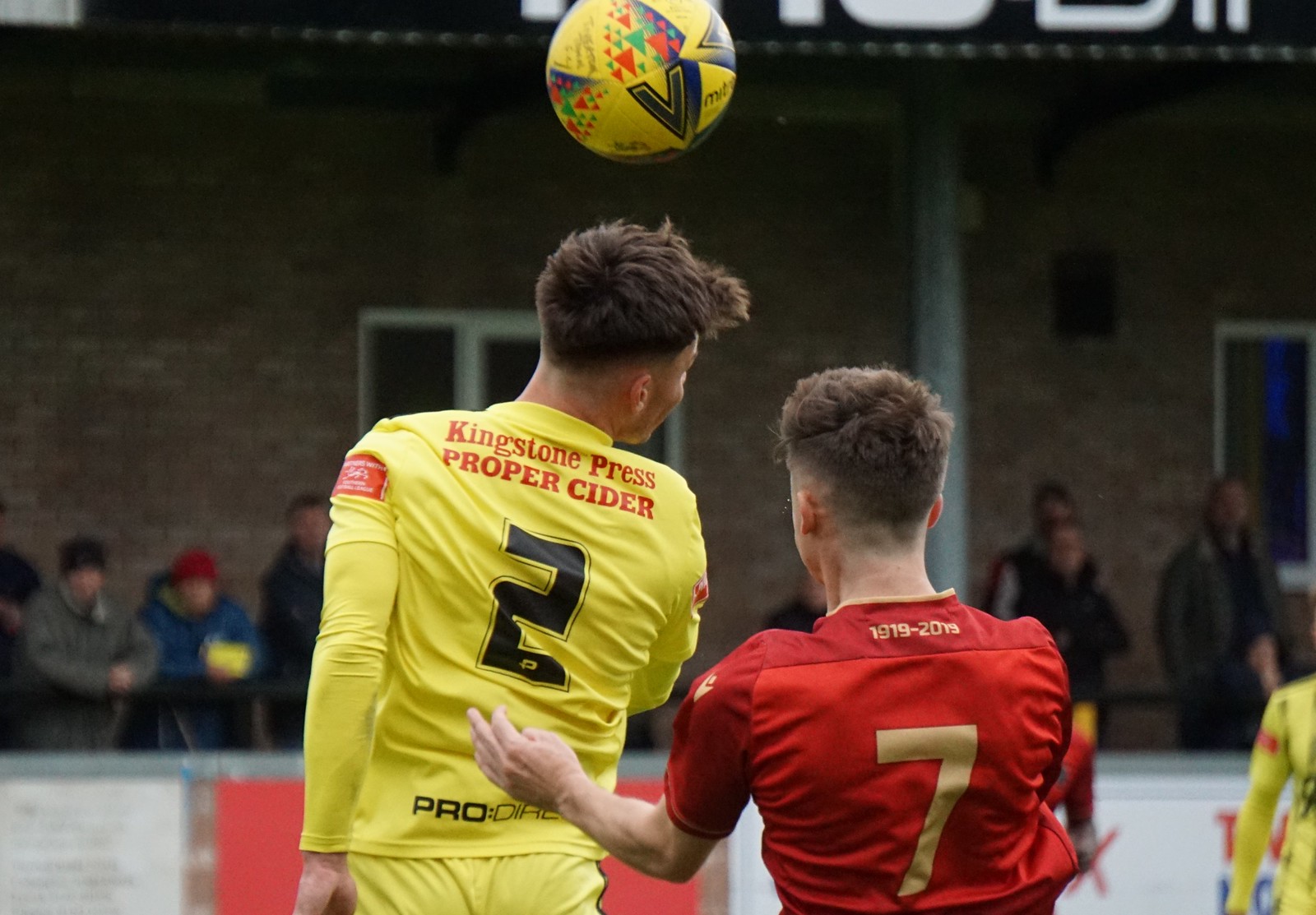This photorealistic image captures an intense moment during a soccer game, focusing on two players in mid-action. The player to the right of center is dressed in a red jersey with a gold number seven on his back, and his short brown hair is slightly ruffled as his left arm is raised. To his left, another player is clad in a yellow uniform with a black number two and "Kingstone Press Proper Cider" printed near the shoulders. This player’s dark brown hair is visible as he tilts his head slightly to the right, both players intent on the action unfolding above them. Suspended in the air above their heads is a striking soccer ball patterned with yellow, red, green, and blue. The background features a blurred crowd of onlookers standing and watching the game in front of a large brown brick building. This action-packed scene vividly captures the dynamic energy of the moment.